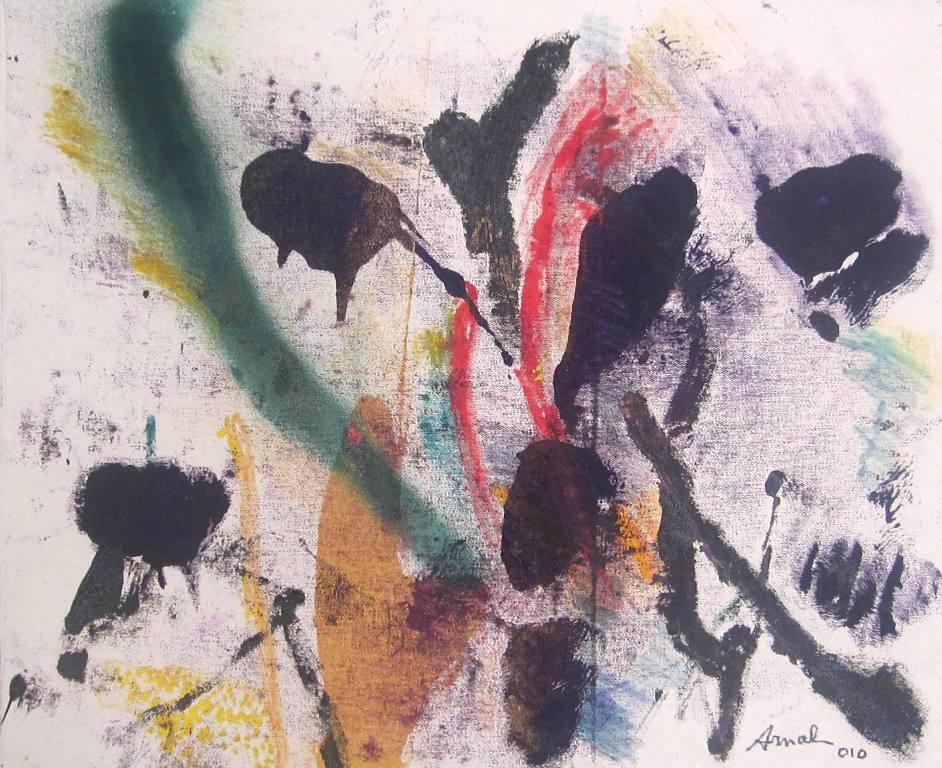The image is an abstract painting with a predominant use of black ink blotches splattered across a primarily whitish or slightly purple background. The black blotches form a concentrated mass down the center and are surrounded by smaller spots and lines. This dark composition evokes a sense of foreboding. In contrast to the black, a large, curved mass of green paint extends diagonally from the top right corner to the center of the canvas, adding a dynamic flow to the piece. Above the central black blotches, two vibrant splatters of red paint emerge, reminiscent of a burst or blood splatter. Scattered throughout are gray rod-like splatters that provide additional texture. 

Hints of yellow and brown paint are subtly incorporated, with the yellow appearing on the left side. The signature of the artist is located in the bottom right corner, reading "A-R-M-A-D-0-1-0" in cursive. The overall chaotic yet deliberate arrangement of colors and forms creates a striking and thought-provoking visual experience.